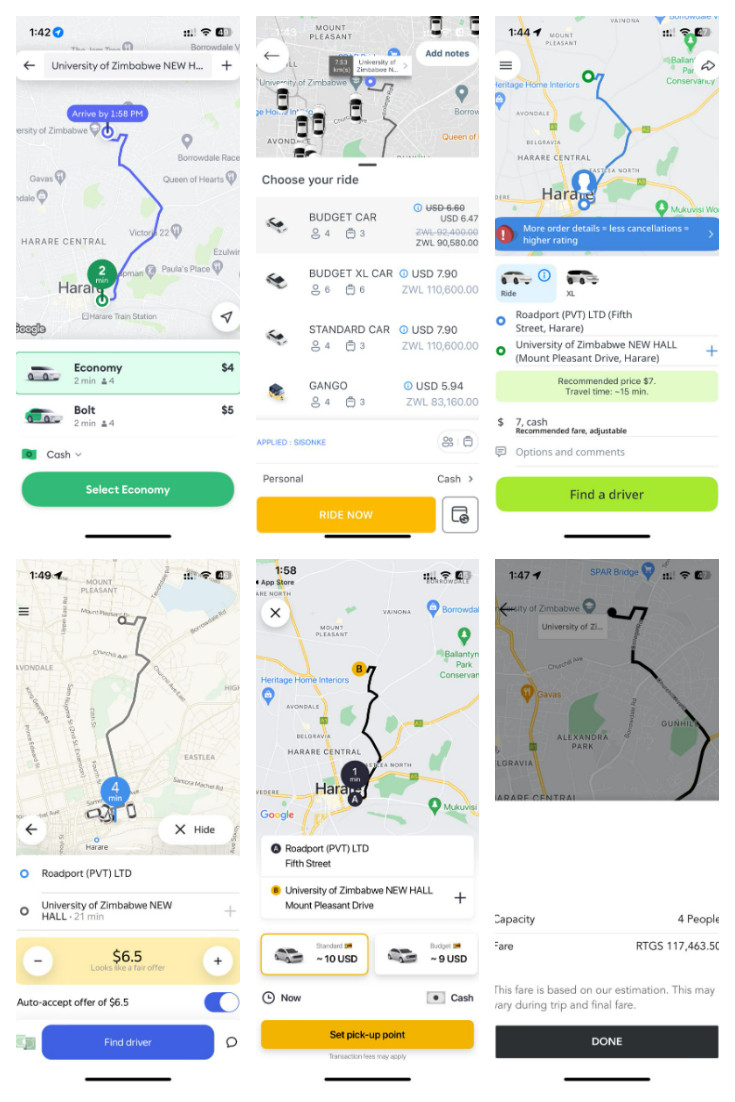The image consists of six different screenshots related to travel and transportation options. 

1. **University of Zimbabwe Navigation**: The first screenshot shows a map with directions from the user's current location to the University of Zimbabwe. The interface includes options for different types of vehicles, displaying two choices.

2. **Budget Car Rental Selection**: The second screenshot features a rental car service, Budget Car, presenting four different vehicle options available for selection.

3. **Destination Location Overview**: The third screenshot depicts the final destination with a map outlining the route to get there. It includes a section titled "Find a Driver" and provides estimated costs for the journey, such as $6, along with driving directions.

Each screenshot is adorned with maps and driving instructions, along with options to select vehicles. Buttons with distinct colors outside of the standard gray text include:
- "Select Economy" button in regular gray
- "Ride Now" button in bright yellow
- "Find a Driver" button in neon green
- "Select Pickup Point" button in mustard yellow
- A final black button labeled "Done"

These interface visuals are designed to help users easily navigate their transportation choices, from selecting vehicle types to pinpointing pickup locations and finalizing their travel plans.